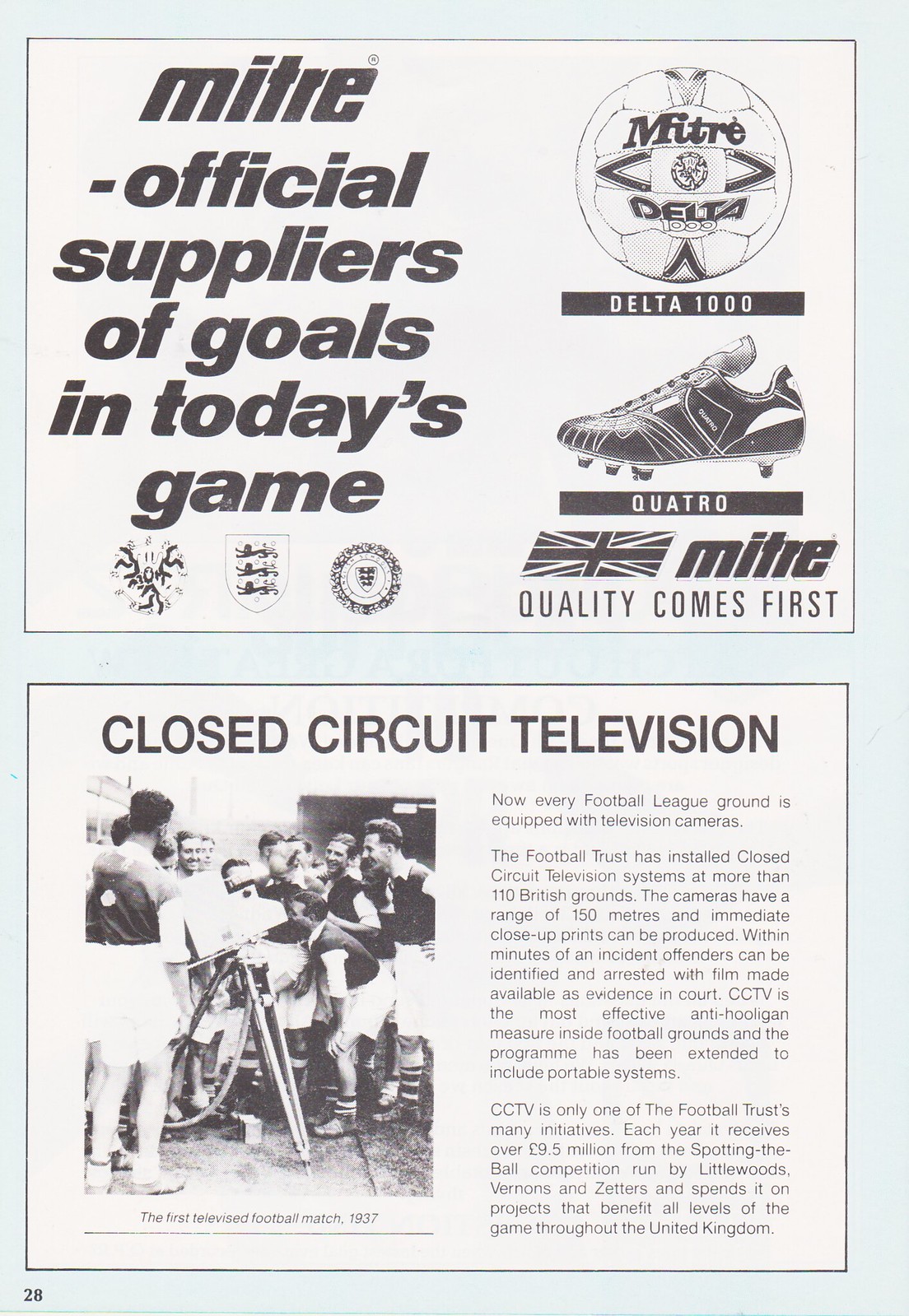The image resembles the end page of a magazine with a very light baby blue background divided into two distinct sections with thin black borders. 

The upper section contains a white box with the bold, black text: "Mitre, official suppliers of goals in today's game". Adjacent to this text, on the right, is a depiction of a soccer ball labeled "MITRE Delta 1000". Below the soccer ball, there’s a black banner with white text that reads "Delta 1000" and situated beneath this is another black banner inscribed with "Quattro", above which are black and white cleats. Further down, the black and white Union Jack is displayed with the text "MITRE quality comes first" in black letters nearby, along with three seals or crests located in the bottom left of the section.

The lower section also contains a white box with a thin black outline and is captioned "Closed-circuit television". This section features a black and white photograph of a group of soccer players wearing black tops and white shorts, huddled together on a grassy field. These players are reportedly watching the first televised football match from 1937 as indicated by the accompanying descriptive text on the right side.